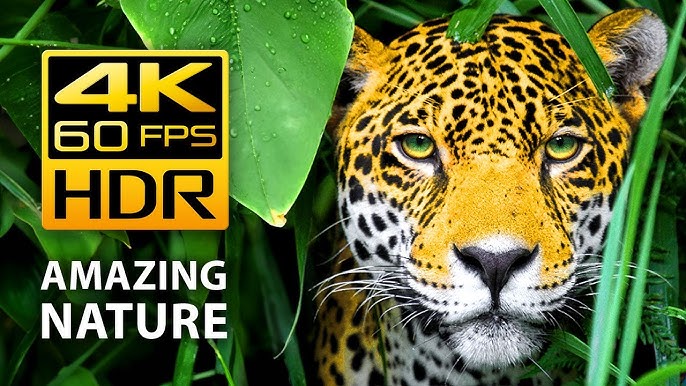An advertising image, twice as wide as it is tall, showcases the stunning capabilities of 4K, 60 frames per second HDR technology. In the upper left corner, a gold square with gold and black lettering highlights these features. Below the square, "AMAZING NATURE" is prominently displayed in bold, all-caps white letters. The background of the image is a vibrant, forested scene featuring large green leaves adorned with glistening raindrops. Dominating the scene is the captivating, direct gaze of a leopard or cheetah. The big cat's striking coat is a mix of yellowish-brown with intricate black spots, contrasted by its white cheeks and throat.